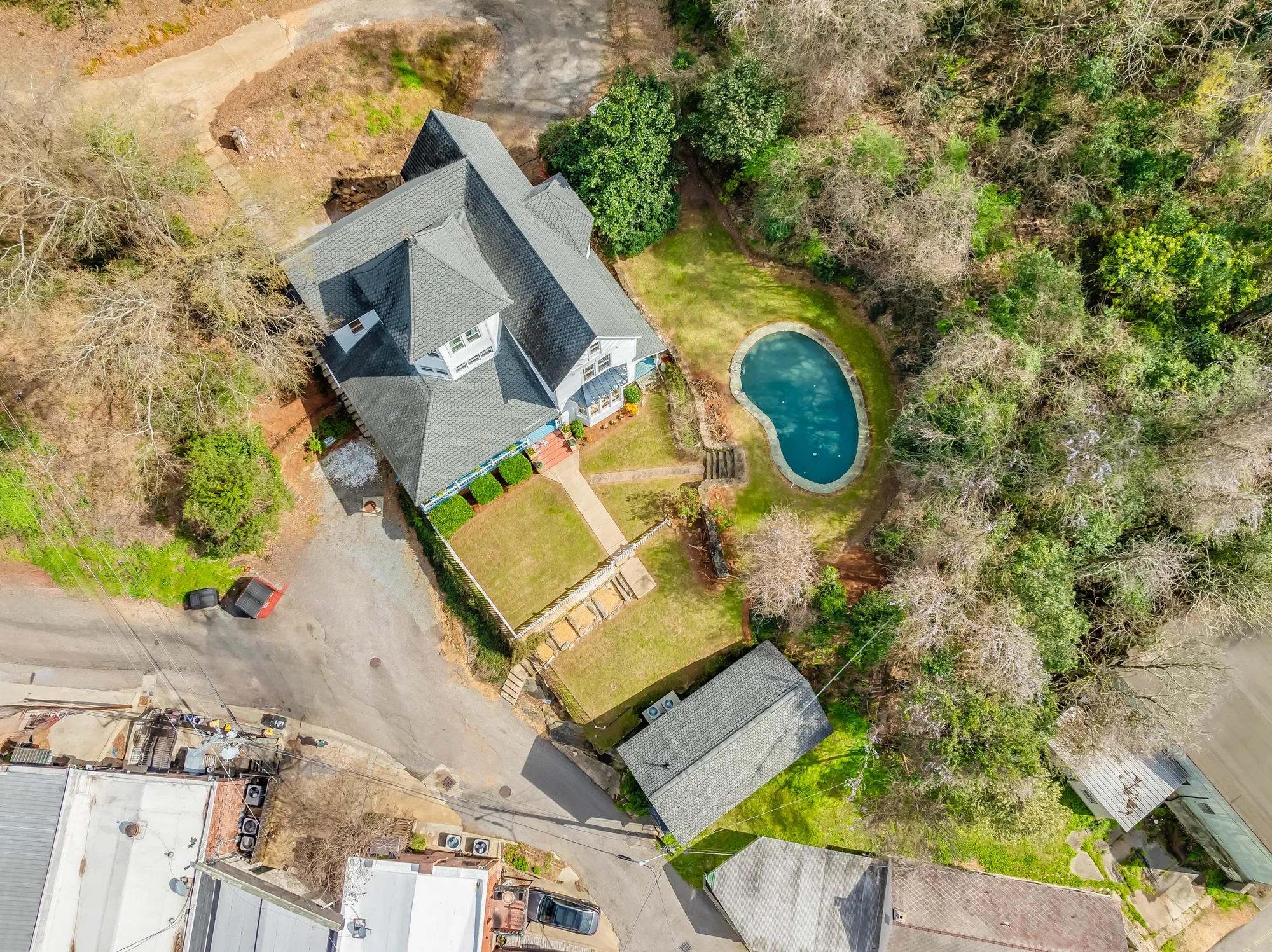The detailed caption for the image is:

An aerial, daytime view of a multi-story house, possibly two or three stories, surrounded by a mix of greenery and dry shrubs. The house features a gray, tiled roof and blue and white siding. From the bird's-eye perspective, the top-level windows are visible, but the lower levels are obscured. A kidney-shaped swimming pool, framed by a gray stone rim, dominates the backyard, which is bordered by a mix of grass, green hedges, and a white picket fence. In front of the house, a walkway leads to the entrance, while the driveway extends to the front and around to the back of the house. To the right, trees and bushes flourish, contrasting with the dried grass around the pool. The property includes additional structures, possibly a garage or guest house, and is surrounded by other properties and roads in a somewhat rural neighborhood. Several vehicles are parked outside, and the sun casts distinct shadows, indicating broad daylight.